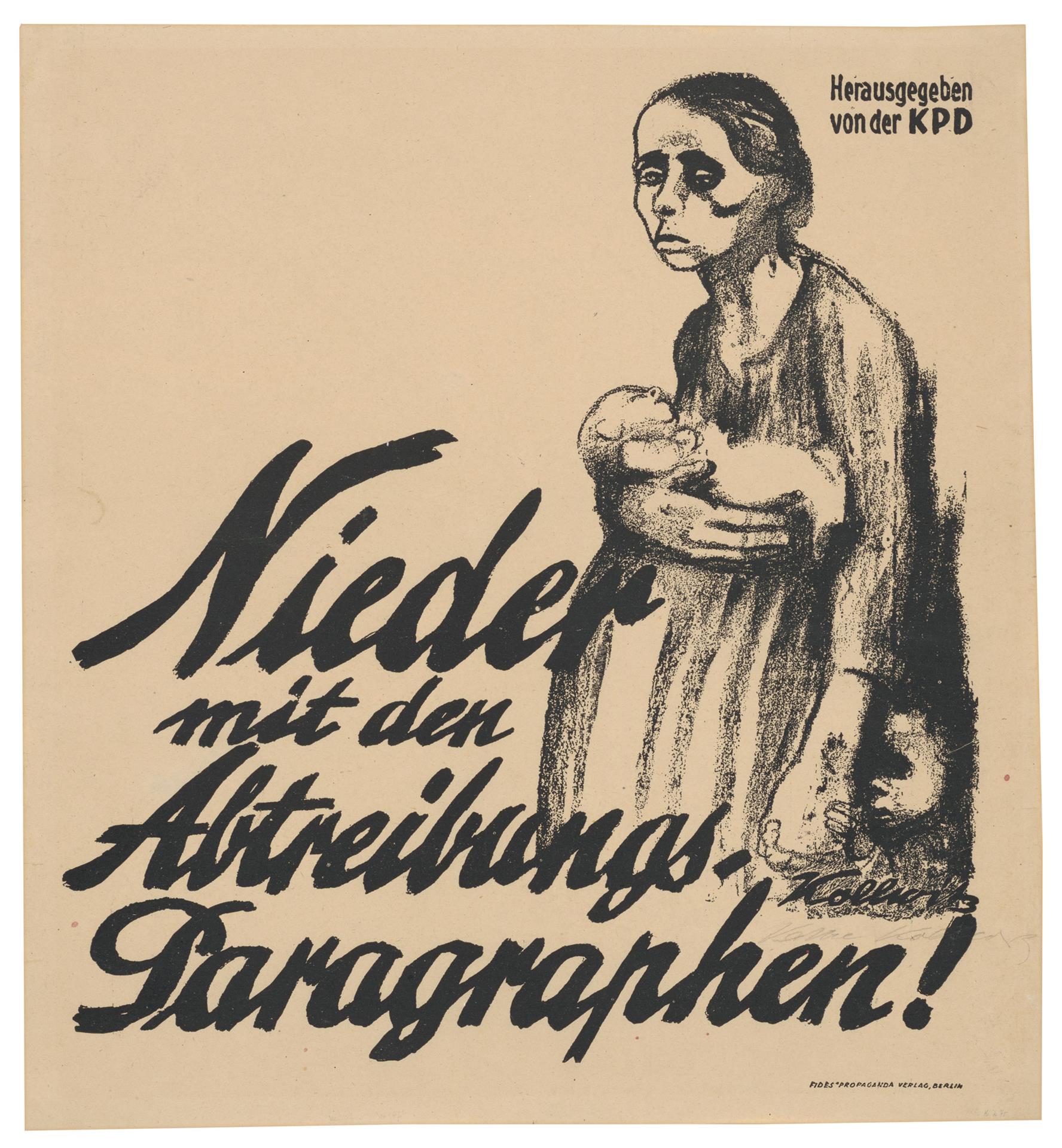The image is a poster with an aged, brown-paper look. It features a detailed black-and-white charcoal illustration of a sad, haggard-looking woman standing in a somewhat slumped-over position, facing towards the viewer. She has dark hair pulled back, with black shading around her eyes, enhancing her sorrowful expression. The woman is wearing a long dress and appears to be carrying a small baby in her right arm, while her left hand holds the hand of a small child standing beside her. The baby and the woman's hand rest against what appears to be either a pregnant belly or postpartum weight. Above the illustration, in the top right corner, there is text in German that reads "Hier gegen den von der KPD." Written prominently across the middle in cursive are the words "Nieder mit den alten Paragrafen," possibly part of an anti-establishment or revolutionary message, rendered in large text. The entire poster is drawn in monochrome, with fine details capturing the emotions and hardship of the depicted woman. There is an unreadable signature and a watermark or copyright notice at the bottom, with the latter being upside down.